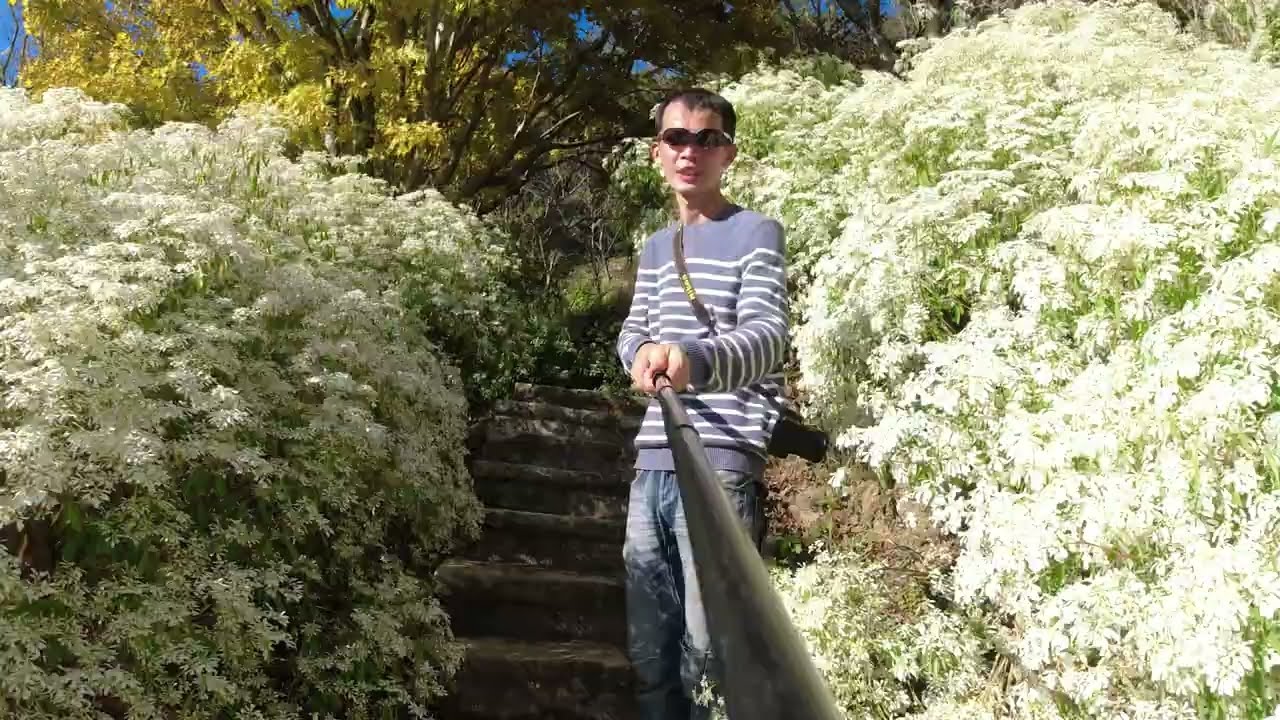The image captures a young Asian man with short, buzz-cut black hair standing on stone steps while holding a selfie stick, taking a picture of himself. The man is dressed in a purple sweater with white stripes and blue jeans. He sports dark sunglasses and has a camera strap slung diagonally across his torso, from shoulder to hip. Surrounding the stone steps are lush green bushes adorned with numerous small white flowers. Further in the background, a sparse tree with green leaves and visible branches adds depth to the scene. The steps appear to ascend a hill, enhancing the sense of a natural, outdoor setting.